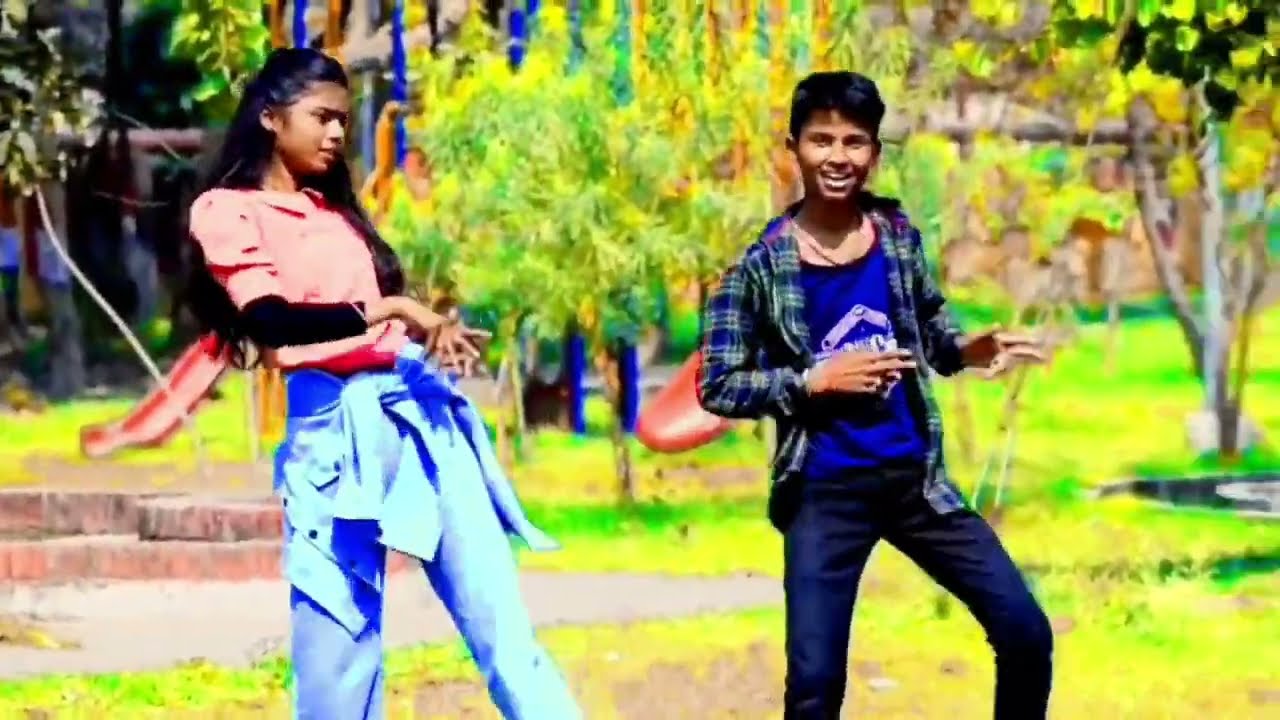In this lively daytime photo, two young individuals stand prominently in a park setting, seemingly engaged in a dance. On the right is a young boy with short black hair and brown skin, smiling openly to reveal his top row of teeth. He is dressed in a blue shirt emblazoned with a white emblem, layered under a long-sleeve blue and green plaid shirt, and dark blue jeans. His hands are raised with two fingers pointing rightwards. To his left is a girl with long black hair cascading down to her waist. She wears a coral shirt ending at her elbows over a black long-sleeve top, blue jeans, and a sweater tied around her waist. Her fingers spread fully as she gestures to the right. The pair, both leaning left with their left legs slightly bent, appear animated and are the photo's focal point. Behind them, the vibrant park features lush yellow and green grass, clusters of trees, and a playground with bright red slides. The lighting suggests the photo was captured during the day.